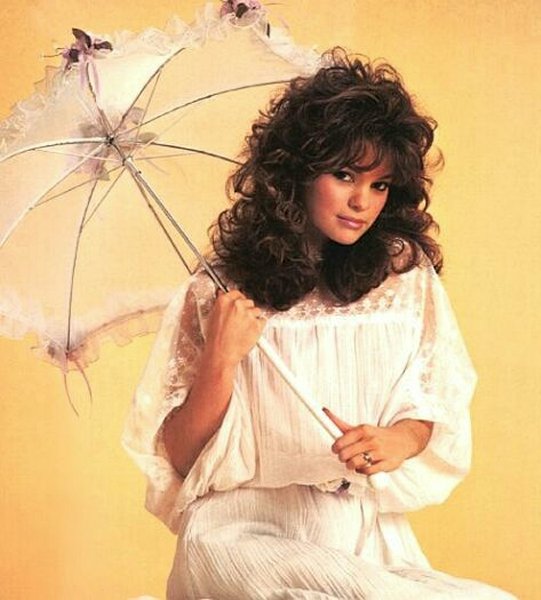This image features actress Valerie Bertinelli posing gracefully against a yellow-beige backdrop. Valerie is seated, draped in a flowing, gauzy white dress adorned with lace detailing around the sleeves, shoulders, and top of the chest. Her medium-length, curly brown hair cascades past her shoulders, framing her face which is highlighted by dark eyes and defined with black eyeliner. In her hands, she holds an ornate, frilly white parasol over her right shoulder, decorated with flowers and bows, resembling an old-fashioned 1800s sun umbrella. The parasol rests on her right shoulder as she supports its weight with both hands, the left one prominently displaying a wedding ring. Valerie's head is slightly tilted, and she gazes upwards, adding an ethereal quality to the portrait.